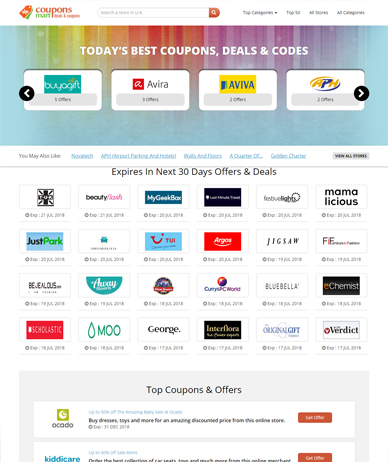The image depicts a webpage from a coupons website. At the very top, there is a white banner. In the upper left corner of this banner, the word "coupons" is displayed in a red font, accompanied by a small red coupon icon to its left. To the right of this red text, there is a search field. Further to the right on the banner are four black menu options, although the text is unreadable due to the small size of the screenshot.

Below the banner, a section titled "Today's Best Coupons, Deals, and Codes" is prominently displayed. This section features four different options, likely representing various companies.

As you scroll down, a black font heading announces "Expires in the Next 30 Days," followed by a list of offers and deals from 24 different companies.

At the bottom of the webpage, the "Top Coupons and Offers" section is visible. Here, you can see logos of the first two companies on the left, with descriptive text about their offers to the right. Each offering is paired with a red button on the far right, presumably for users to click and access the deal. Due to the screenshot's small size, the exact text on the red button is unreadable.